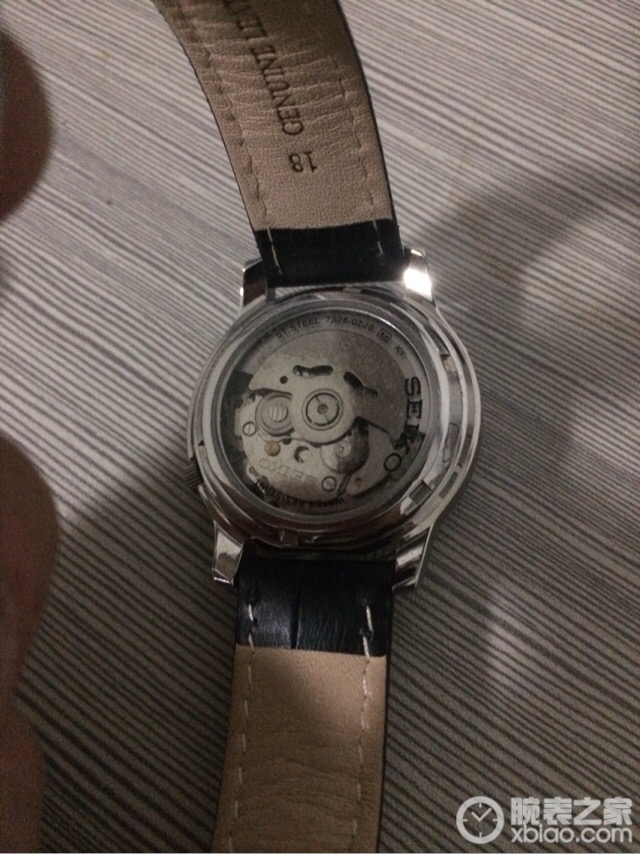This detailed photograph captures the reverse side of a Seiko wristwatch, meticulously displayed upside down on a wooden table. The wood grain texture of the table background adds a warm, organic contrast to the intricate mechanics of the watch. The watch band, made of genuine leather, is open and positioned to face away from the camera. The inner side of the band is a natural tan color with black edges, suggesting that the outer side, which would be visible when worn, is fully black. Imprinted on the leather strap is the designation "18 Genuine LEA," verifying its authenticity. The bottom of the watch case reveals its complex inner mechanics, showcasing an array of tiny gears, circles, and dials, hinting at the precision and craftsmanship behind its construction.